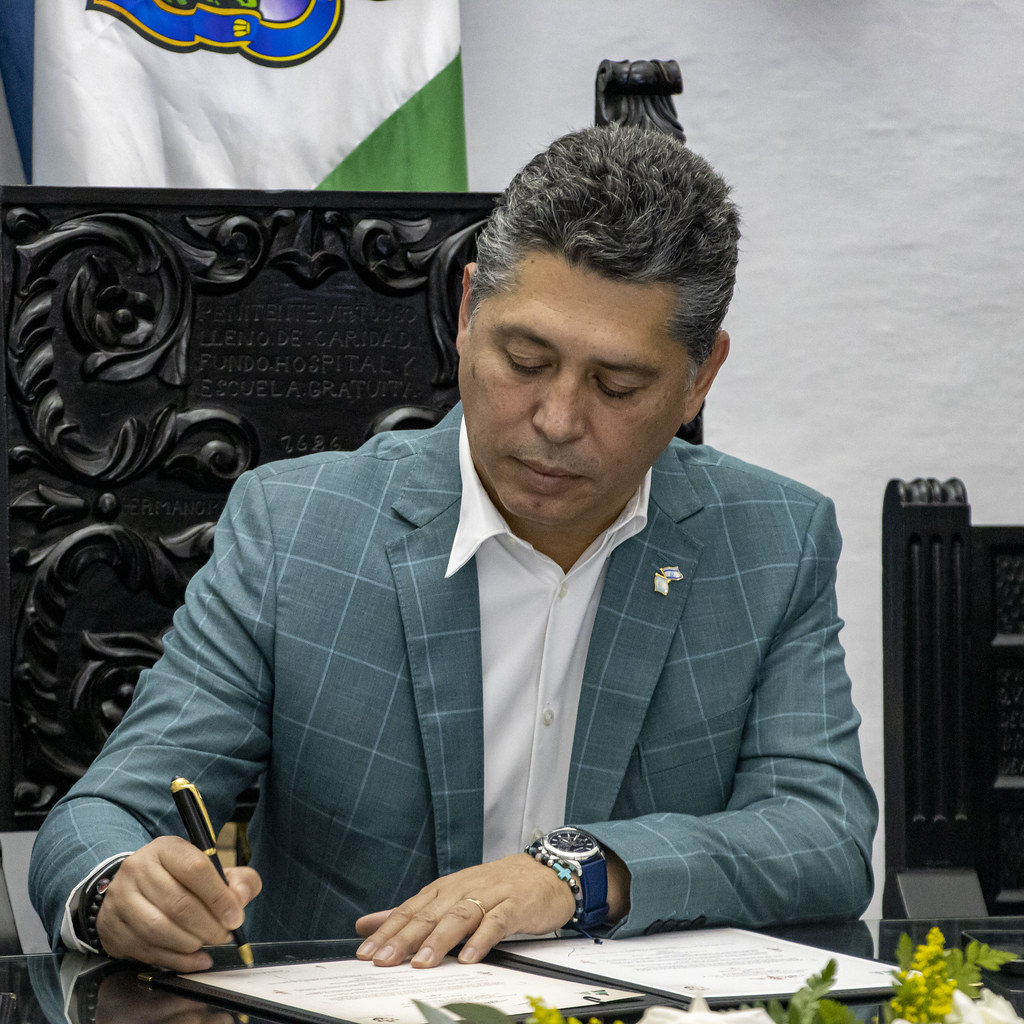In this detailed image, a man with black and silver hair is seated at a desk, engrossed in signing a couple of documents on a glass-topped table. He is wearing a light blue jacket adorned with white stripes crossing in a checkered pattern, over an open-collared white button-down shirt. A blue watch and a beaded bracelet embellish his wrists, while a small, unidentified pin decorates his left lapel. The man is seated comfortably in a black chair featuring intricate wooden carvings. Behind him, to the left, there is a flag bearing green, white, and a blue emblem. The backdrop consists of a plain, grayish-white wall, adding a neutral contrast to the scene's elaborate details.